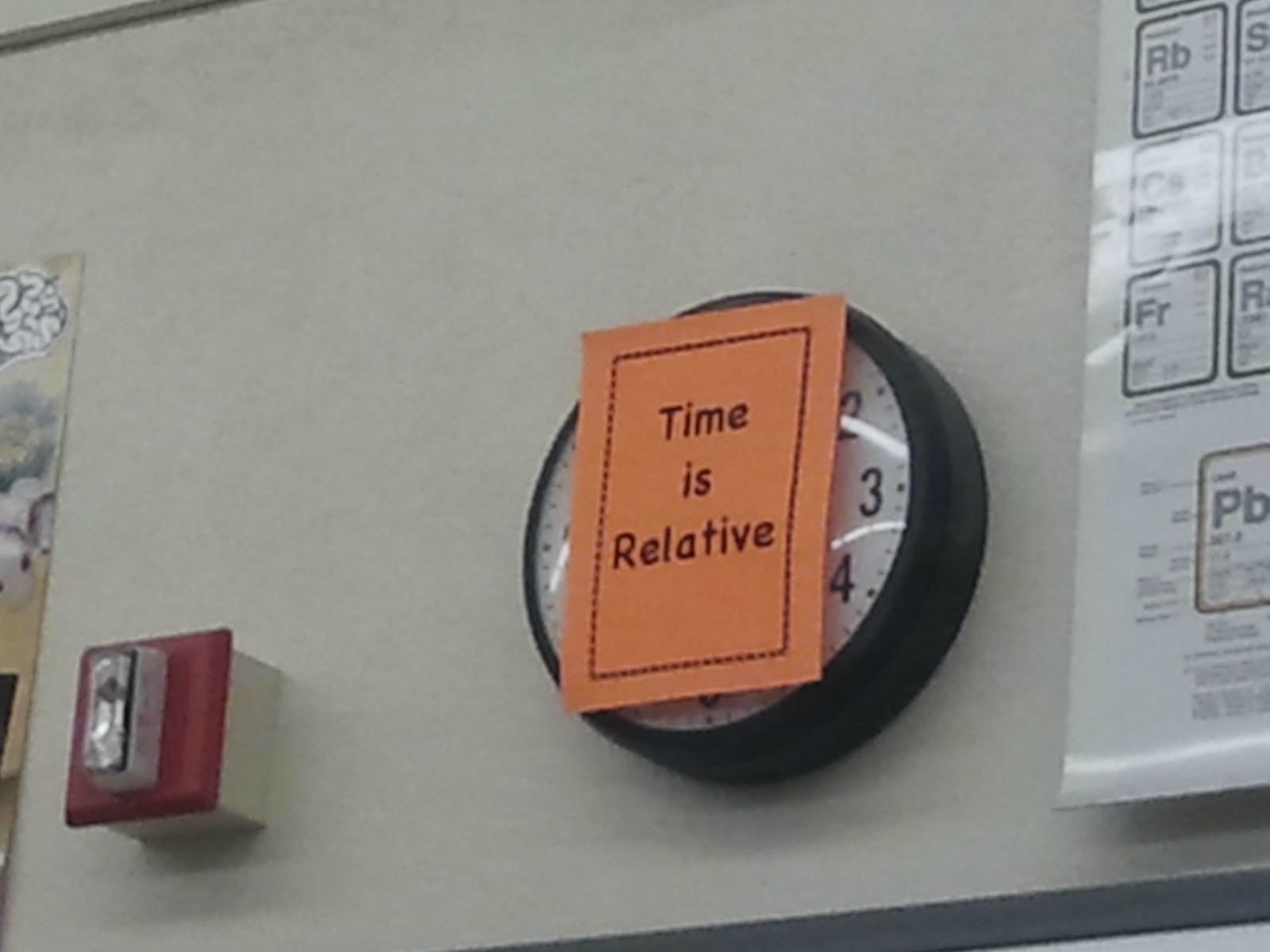This image depicts a science classroom wall with a tan background featuring a notable round black-bordered clock with a white face. The clock displays the numbers 2, 3, and 4, but the hands are obscured by an 8.5 x 11-inch orange sheet of paper taped to the front. This paper has a black dotted-line rectangle framing the phrase "Time is relative." To the left of the clock, there is a red fire alarm box with a blinking light. To the right, part of a periodic table poster is visible, showing elements such as FR, PB, and RB. The setting suggests a meticulously arranged learning environment, likely designed by a physics teacher to evoke curiosity among students.